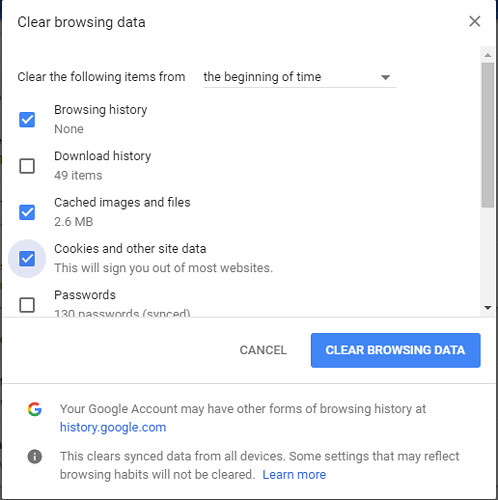A web browser settings page is displayed, highlighting various options for clearing browsing data. At the top of the image, the title "Clear browsing data" is prominently written in black. Beneath this heading, a list of data types is shown. 

First, the "Browsing history" option is checked in blue, indicating it will be cleared, though it states there are "None" under browsing history. Next is the "Download history" option, which shows "49 items." Following this, "Cached images and files" are listed, amounting to "2.6 megabytes."

The "Cookies and other site data" option comes next, with a warning that clearing this will sign the user out of most websites. This is followed by the "Passwords" option indicating "130 passwords synced."

To the right of these options, the "Clear Data" button is prominently highlighted in white against a blue background, ready for activation.